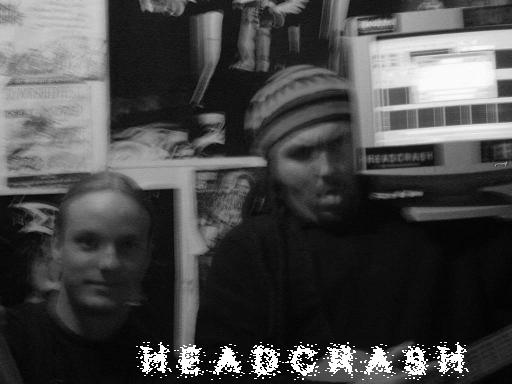The photograph, likely from an album cover or CD cover, is a black-and-white and slightly out-of-focus image embodying a 90s grunge rock aesthetic. Central to the image are two male individuals, with the man on the right appearing taller and donning a patterned beanie and black hoodie, his expression seemingly angry. The man on the left, who has light hair slicked back and is wearing a dark shirt, directly faces the camera while making a silly face with his tongue out. Both are seated in front of a background that includes a computer monitor on the right side and shelving with various unidentifiable items. The photograph features a bold, deteriorating white spray-paint style text at the bottom that reads "HEADCRASH," indicating the name of the band, which also appears faintly on the computer monitor. The overall composition and typography reinforce the edgy and raw vibe typical of the era’s grunge rock scene.